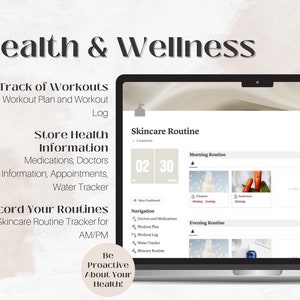This image seems to be a partial screenshot of a flyer or website focused on health and wellness. The heading "Health and Wellness," with the 'H' cut off, stands prominently at the top. The design features a sophisticated gray and cream-colored background. Below the heading is a list, with "Track Workouts" appearing in bold text, followed by "Workout Plan" and "Workout Log" in a lighter, less bold font.

Further down, the text outlines various features, including "Store Health Information," "Medications," "Doctor Information," "Appointments," and "Water Tracker," each separated by commas. The cut-off section below these suggests additional functionalities related to health tracking. Visible text includes "cord your routines," hinting at "Record your routines" and a "Skin care routine tracker for a.m./p.m."

Prominently featured within a brown circle, the text "Be proactive about your health" encourages proactive health management. To the right, there is an image representing a likely computer interface for a skin care routine tracker. This interface showcases different icons for morning and evening routines, labeled "Navigation," with several clickable menu options.